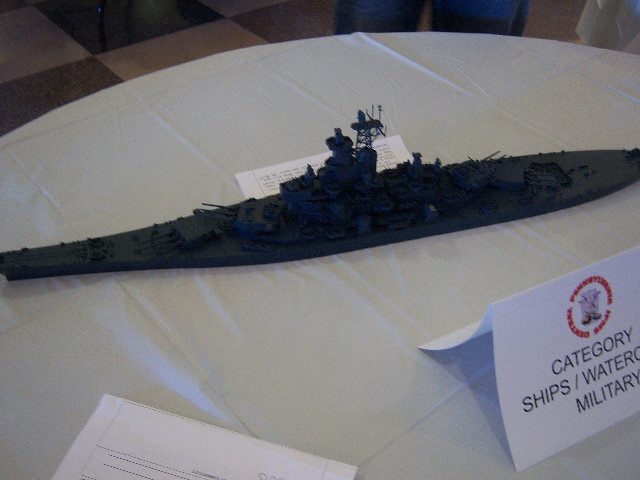The image is a horizontal, rectangular photograph likely taken in a military museum showcasing a model of a Navy destroyer on a round table covered with a slightly wrinkled white tablecloth. The model ship, characterized by its long, narrow shape with towers, antennas, radar systems, and turrets, appears completely black, obscuring finer details due to the dark lighting. Prominently displayed at the front right corner of the table is a small, folded info card with the text "Category: Ships/Water...Military," adorned with a red circle and logo above the text. Another indistinct card is on the lower left side of the table. In the dimly lit background, a patterned carpet or tile floor, possibly checkerboard, and some indistinguishable objects add to the setting’s ambiance.